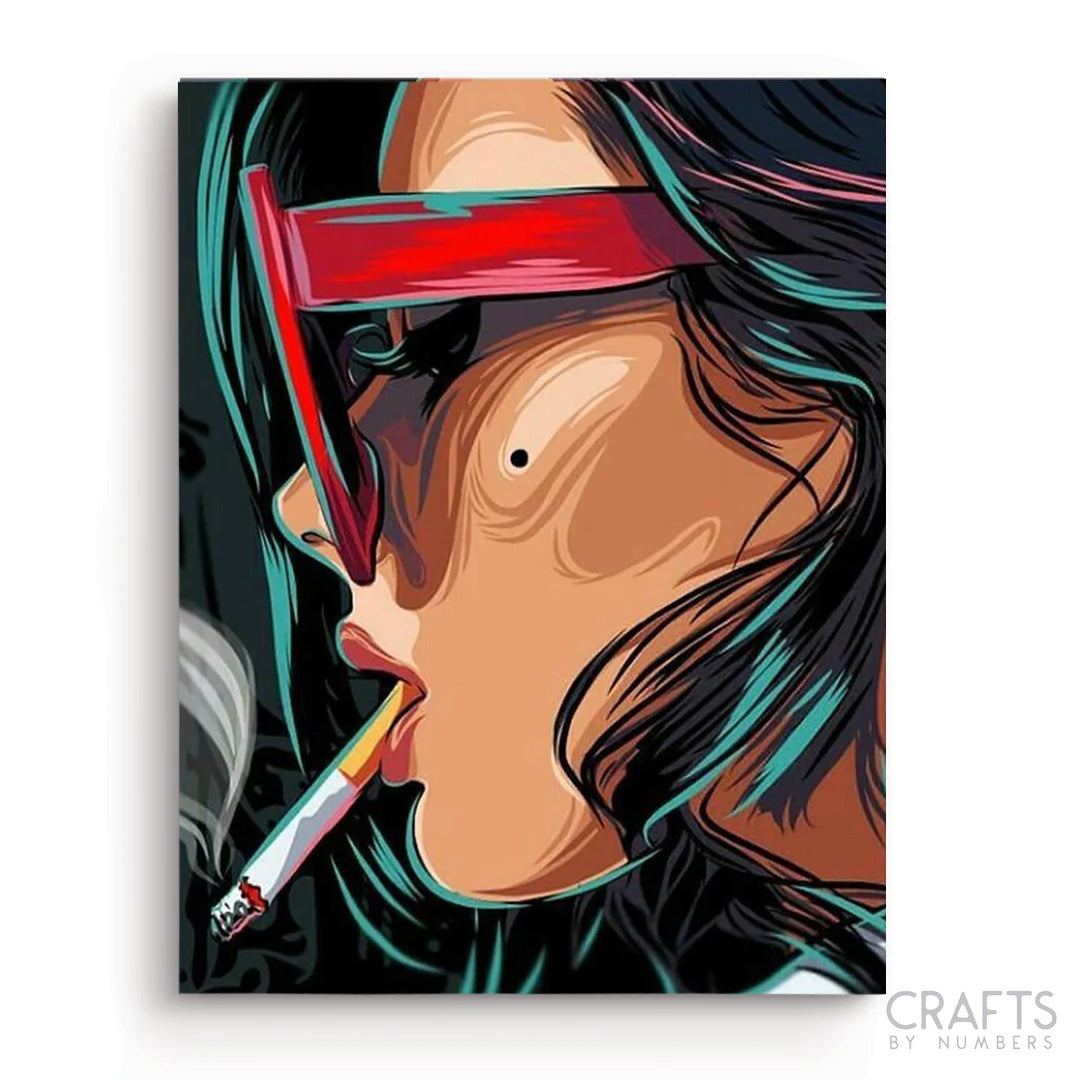The image features a digital pop art style side profile of a woman facing left, created using computer graphics and possibly part of an art kit titled "Crafts by Numbers." The woman has medium-length light green hair with touches of pink, particularly visible at the top right of the image. Her hair merges seamlessly into the background. She is wearing red sunglasses and has pronounced, long, and curled eyelashes. A lit cigarette dangles from her mouth, complemented by her red lipstick. She also sports a black circular mole on her left cheek, adding a distinctive detail to her look. The overall color palette includes tan for her skin tone, red for her lips and glasses, and black accents.